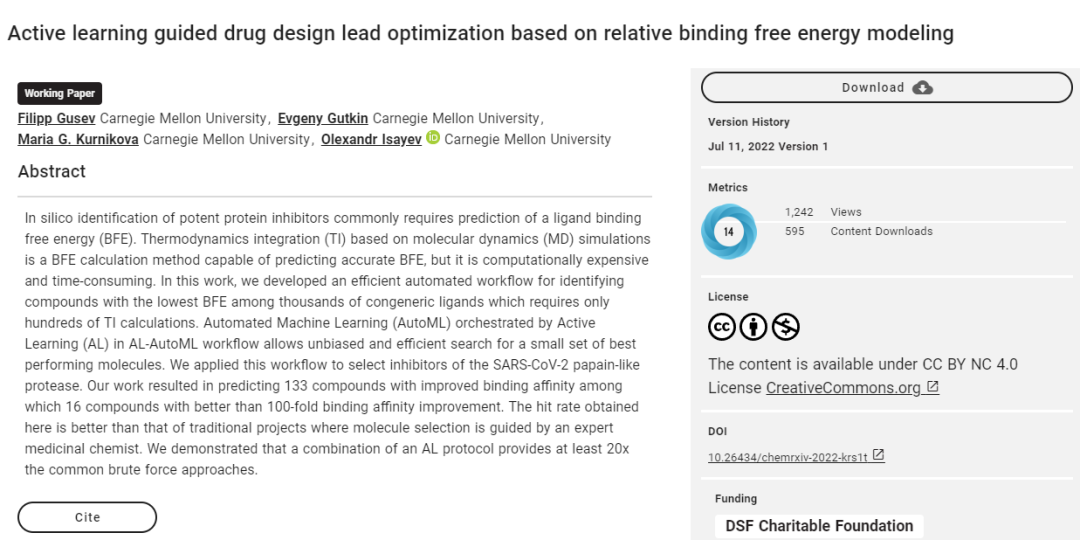The website page displayed prominently features a black header on a white background with the title "Active Learning Guided Drug Design Optimization Based on Relative Binding Free Energy Modeling" written in black text. Below the title, there is a black tab labeled "Working Paper" in white text. The authors listed include Philip Lipp (Carnegie Mellon University), Yousef Gusev (Carnegie Mellon University), Evgeny Kokkin (Carnegie Mellon University), Maria G. Karnikova (Carnegie Mellon University), and Alexander Isaev (Carnegie Mellon University).

The page continues with an abstract of the article, initiating the body of the text. Towards the bottom of the web page, a bordered section displays the word "SITE" in capital letters at the center, with a capital ‘C’.

Adjacent to this section, a gray background features an oval button at the top that says "Download" in the center, accompanied by an icon of a cloud with a down arrow. Below this, the text outlines the version history noting, "June 11, 2022, Version 1". The section provides metrics such as views, content, downloads, license information, DOI, and funding. Lastly, the page mentions "DSF Charitable Foundation" on a white background in capital letters under the funding section.